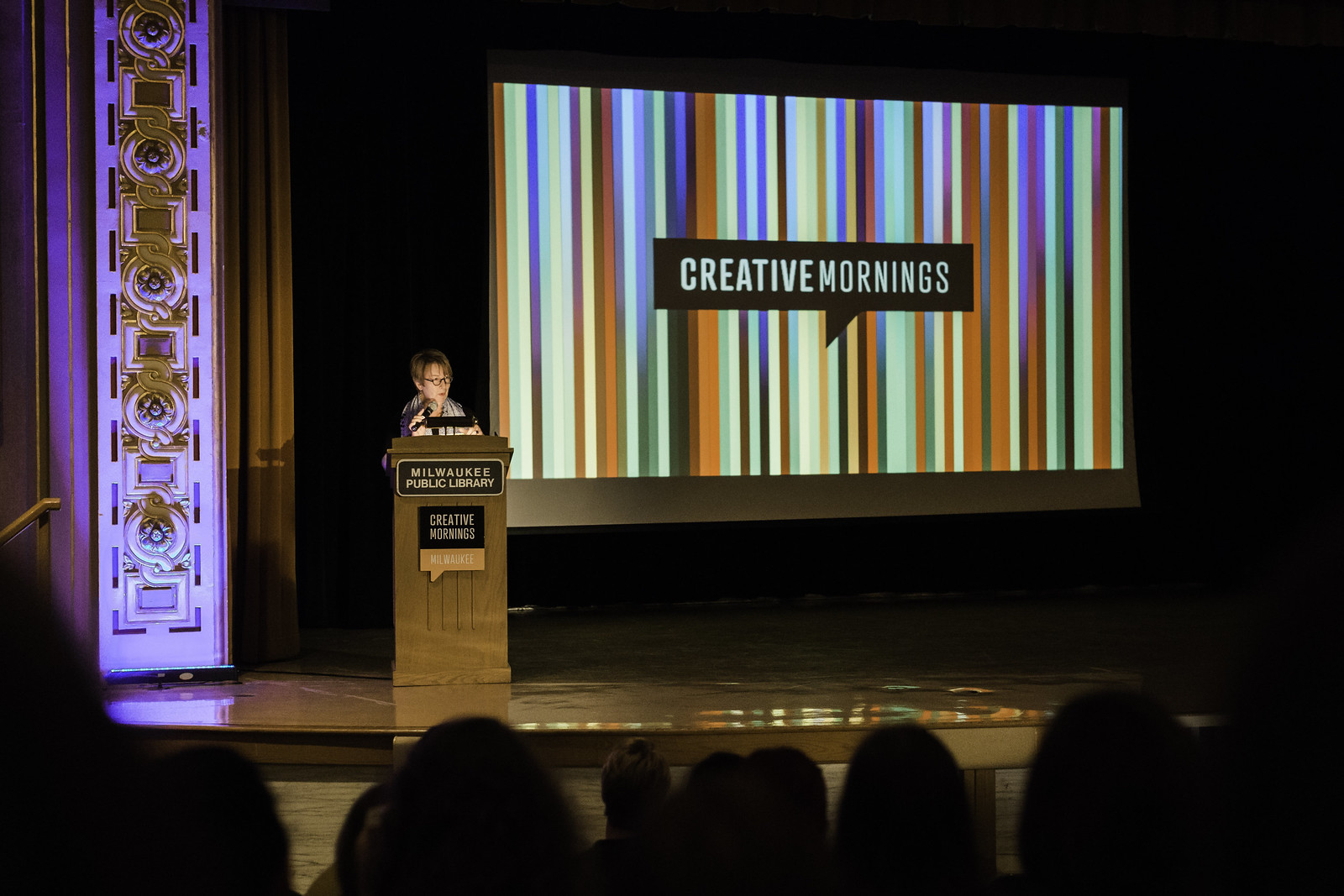In a dimly-lit auditorium, a poised woman stands at a podium on a brightly illuminated stage, addressing an attentive audience. The podium, adorned with the words "Milwaukee Public Library Creative Mornings," is flanked by a large projector screen displaying vibrant, multicolored stripes that mirror the hues of the speaker's shirt. Both the screen and podium proudly bear the "Creative Mornings" and "Milwaukee" branding. The stage features intricate tile work, evoking the grandeur of a theater more than a library, adding a unique backdrop to the scene. At the podium, the woman is equipped with a microphone and a reading light, ensuring her voice and presence command the room during the event.